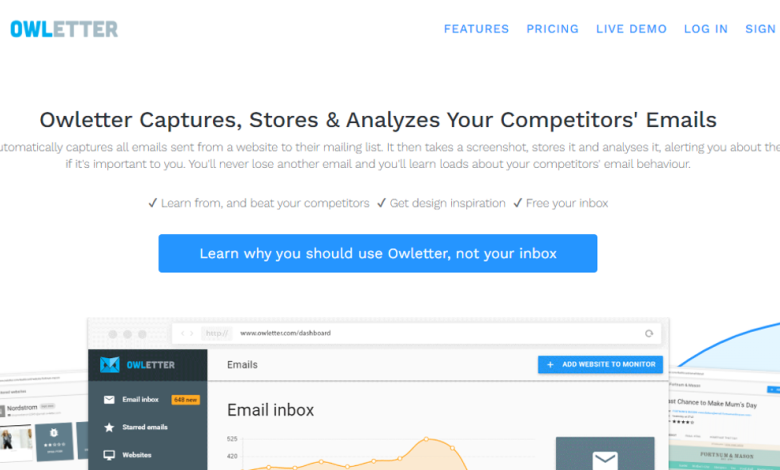In this landscape-mode screenshot set against a white background, the upper left-hand corner prominently features the name "OWLletter". The "OWL" segment is distinguished in bold blue letters, while "ETTER" appears in muted gray. On the upper right-hand side, small blue capital letters list navigation options: Features, Pricing, Live Demo, Login, and Sign.

Below, a bold black headline announces, "OWLletter captures, stores, and analyzes your competitor's emails." Directly beneath this headline, a small gray text elaborates: "Automatically captures all emails sent from a website to their mailing list. It then takes a screenshot, stores it, and analyzes it, alerting you about the...," ending abruptly as the text is cropped.

Further down, the benefits of using OWLletter are encapsulated in three succinct phrases, each preceded by a gray check mark: "Learn from and beat your competitors," "Get design inspiration," and "Free your inbox." 

A lengthy, narrow blue rectangle below these phrases contains white text that invites users to "learn why you should use OWLletter, not your inbox." Beneath this call-to-action, a series of OWLletter screenshots are displayed, offering a visual glimpse into the platform's interface and capabilities.